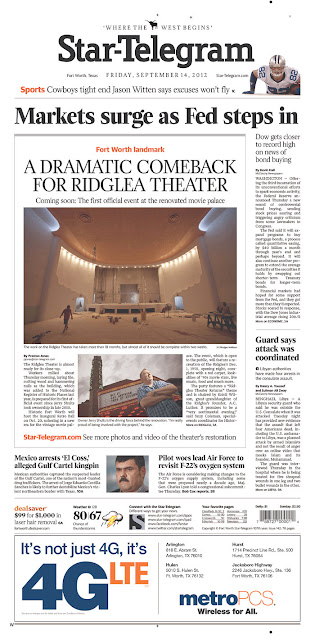The image depicts the front page of the "Star-Telegram," dated Friday, September 14, 2012, with the headline "Where the West Begins" prominently displayed. Below, in large black letters, is the newspaper's title, "Star-Telegram." Featured prominently in red is the sports headline: "Cowboys Tight End Jason Witten Says Excuses Won't Fly," accompanied by a photo of a football player in a white uniform with blue numbers and a silver helmet.

In another section, the headline "Market Surge" is noted, followed by "Step In," discussing a Fort Worth landmark: a dramatic comeback for the Ridley Theater. An image shows a person in a blue and white checkered shirt standing outside the theater, with a caption about the first official event at the newly renovated movie palace.

Additional headlines include "Dell Gets Closer to Record High on News of Bond Buying" and "Guard Says Attack Was Coordinated." Lastly, an article's heading mentions "Mexico Arrests Alleged Gulf Cartel Kingpin," alongside a note about the Air Force revisiting its oxygen system.